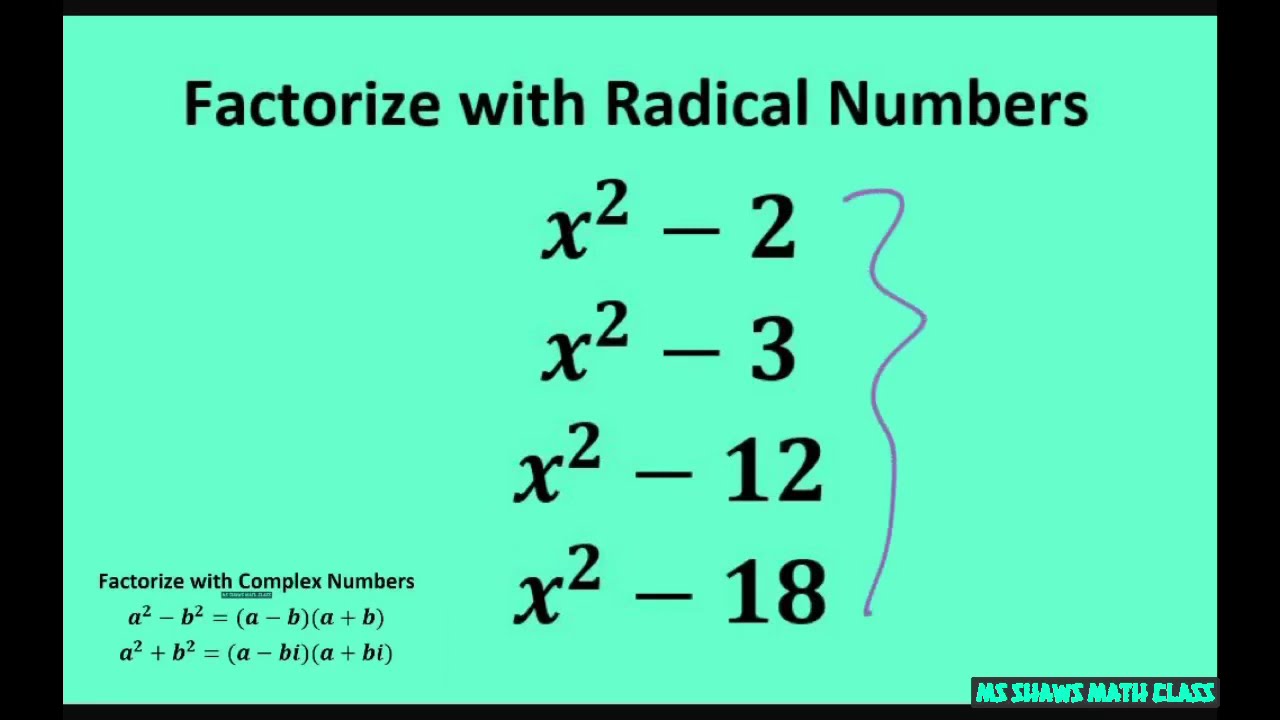This image, likely a screenshot or a note card intended for a math class, is framed with a black border, appearing thicker on the vertical sides. The background boasts a bright seafoam green color. The prominent heading at the top reads "Factorize with Radical Numbers" in black print. Below this, four rows display different equations: X² - 2, X² - 3, X² - 12, and X² - 18. To the right of these equations is a squiggly line, possibly drawn in pink or blue. Positioned in the lower-left corner, the text "Factorize with Complex Numbers" introduces two formulas: a² - b² = (a - b)(a + b) and a² + b² = (a - bi)(a + bi). The lower-right corner features the label "Ms. Shaw's Math Class."